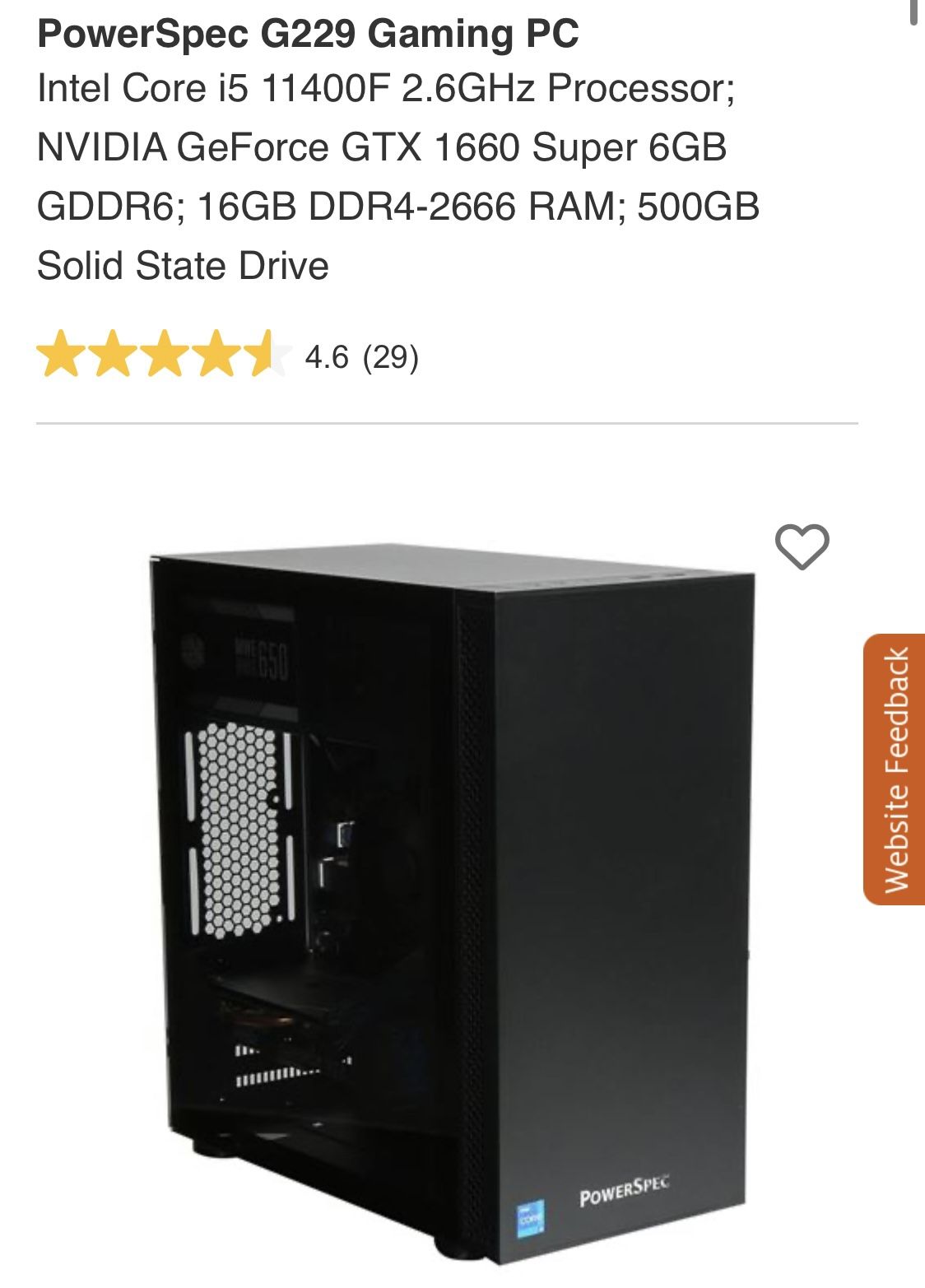The PowerSpec G229 Gaming PC features an Intel Core i5-11400F 2.6 GHz processor, coupled with an NVIDIA GeForce GTX 1660 Super 6GB GDDR6 graphics card. The system comes equipped with 16GB of DDR4-2666 RAM and a 500GB solid-state drive. The case of the PC is constructed from sleek black metallic material. The back of the case includes a vent for optimal airflow, while the sides are unadorned with any visible components. The front of the case is minimalist in design, featuring a flat black surface. On the left side, there is a distinctive blue square and accompanying text that reads "PowerSpec." The machine stands on rubber feet, ensuring stability and reducing vibration. The overall build and specifications indicate a robust gaming performance, with the product rated 4.5 stars out of 5 by 29 reviewers.